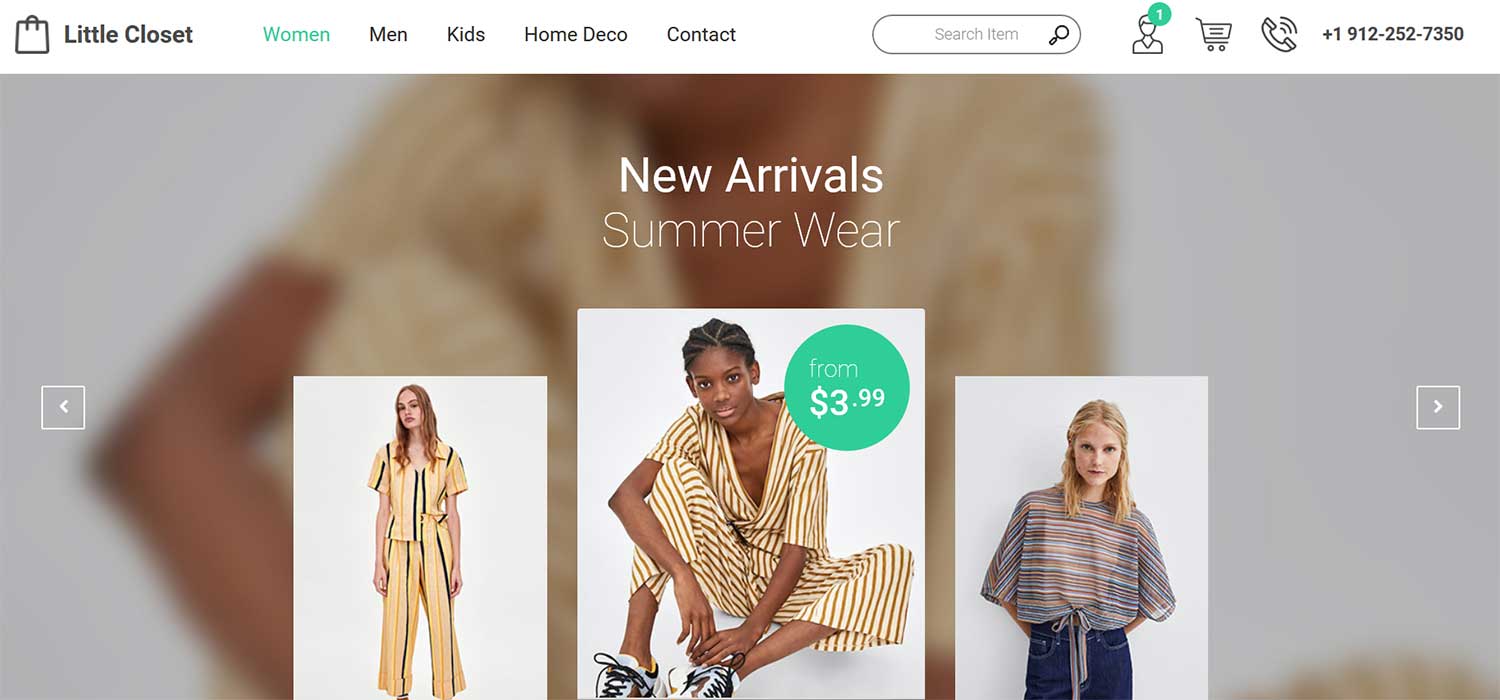Screenshot of an e-commerce website called "Little Closet." On the top left corner, the "Little Closet" logo, depicted as a shopping bag, is prominently displayed. Adjacent to the logo are five navigation tabs labeled: "Women" (highlighted in green to indicate the current section), "Men," "Kids," "Home," and "Deco," followed by a "Contact" link, with small spaces separating each tab. Positioned next to these tabs is a search bar for users to easily find products. To the right of the search bar are three icons: a message icon, a shopping cart icon, and a call icon, alongside the customer service number, 912-252-7350.

The main content area of the web page features a section titled "New Arrivals Summer Wear" showcasing three images. The central image highlights an African-American model dressed in a striped, pajama-like summer dress. A green circle overlaying this picture indicates the price starting "from $3.99." The other two images on either side feature white models standing against a pristine white background, presenting additional summer wear options.